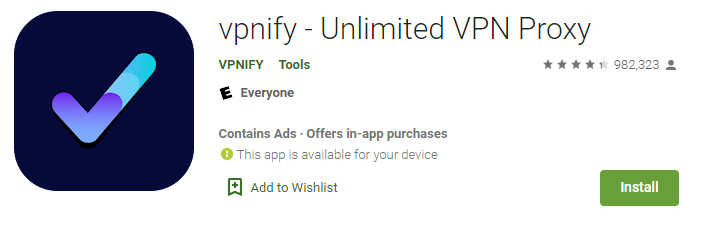The image is an app listing for "VPNify - Unlimited VPN Proxy," designed for installing a VPN service. The layout is horizontally elongated with key details organized across the screen. 

On the left side of the image, there is a prominent black box featuring a checkmark that is a blend of purple and two shades of green. 

The right side showcases the app's name "VPNify - Unlimited VPN Proxy" against a white background, with "Vinipy Tools" written below it. To the right of the app name, a rating of 4.5 stars is displayed alongside a review count totaling 982,323. 

Additionally, there's an "E for Everyone" rating label on the left side, and text indicating that the app "contains ads" and "offers in-app purchases."

Beneath this, a green circle with a white eye icon signifies the app's availability for the user's device. Following that, there's a ribbon outlined in green with a green plus sign inside, labeled "Add to your wish list," and to the right of this, a green "Install" button with white font for immediate downloading.

The color palette includes black, purple, two shades of turquoise green, white, gray, and olive green.